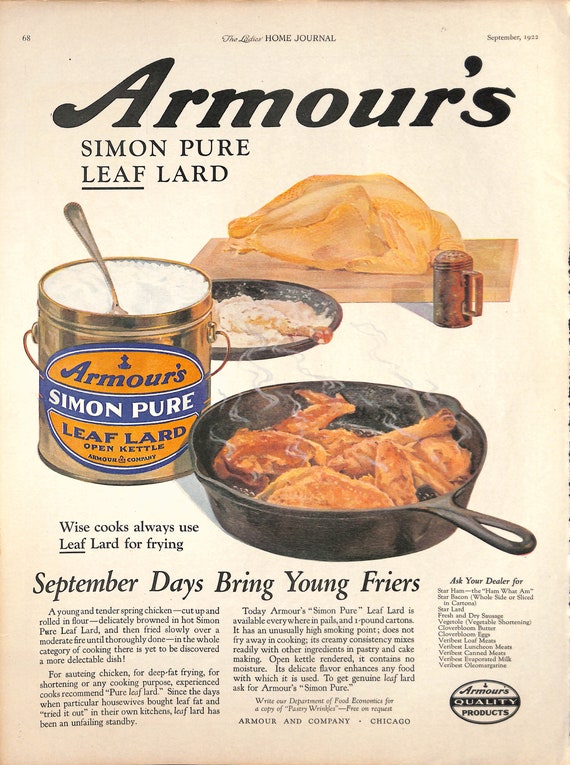This vintage advertisement poster from *The Ladies' Home Journal*, September 1923, features a meticulously staged scene showcasing a premium cooking product, Armour’s Simon Pure Leaf Lard. The ad headline in bold black letters, "Armour’s Simon Pure Leaf Lard", highlights the product, with "Leaf" prominently underlined in the title within an orange circle, emphasizing its purity. 

The visually appealing poster depicts a wholesome culinary process. At the top center, there's an image of a whole chicken on a wooden cutting board, positioned next to a salt or flour shaker. Below this, the ad distinctly shows the chicken being prepared: a leg is dipped in a bowl of white flour. Adjacent to this, an iconic image of chicken pieces frying to a golden brown in a cast iron pan catches the eye. Beside the pan, a can of Armour's Simon Pure Leaf Lard is displayed, illustrating the product in a pail, emphasizing its creamy consistency and its high smoking point.

The detailed textual content illustrates culinary expertise: "Wise Cooks Always Use Leaf Lard for Frying. September Days Bring Young Fryers." This phrase pairs with an extended description of the meticulous cooking method, highlighting the use of young, tender spring chicken pieces, rolled in flour, browned delicately in hot Simon Pure Leaf Lard, and fried slowly over a moderate fire. The text underscores the product's long-standing reliability since "the days when particular housewives brought leaf fat and tried it out in their own kitchen".

Furthermore, the advertisement highlights the versatile usage of the lard for saucing chicken, deep fat frying, shortening, and other cooking purposes, noting its high smoking point and how it does not fry away. The included traditional family tips enhance its appeal, alongside a prompt to request a free copy of "Pastry Wrinkles" from Amherst Company, Chicago, accentuating the product's credibility.

Additionally, the ad includes mentions of other products under the brand, such as "Clover Bloom Butter and Eggs, Verbatim Loaf Mix, and Verbatim Canned Meat," aligning with the Armour Quality Products logo at the bottom. This richly detailed ad serves as both a visual and textual testament to the product's long-standing reputation and quality in cooking.